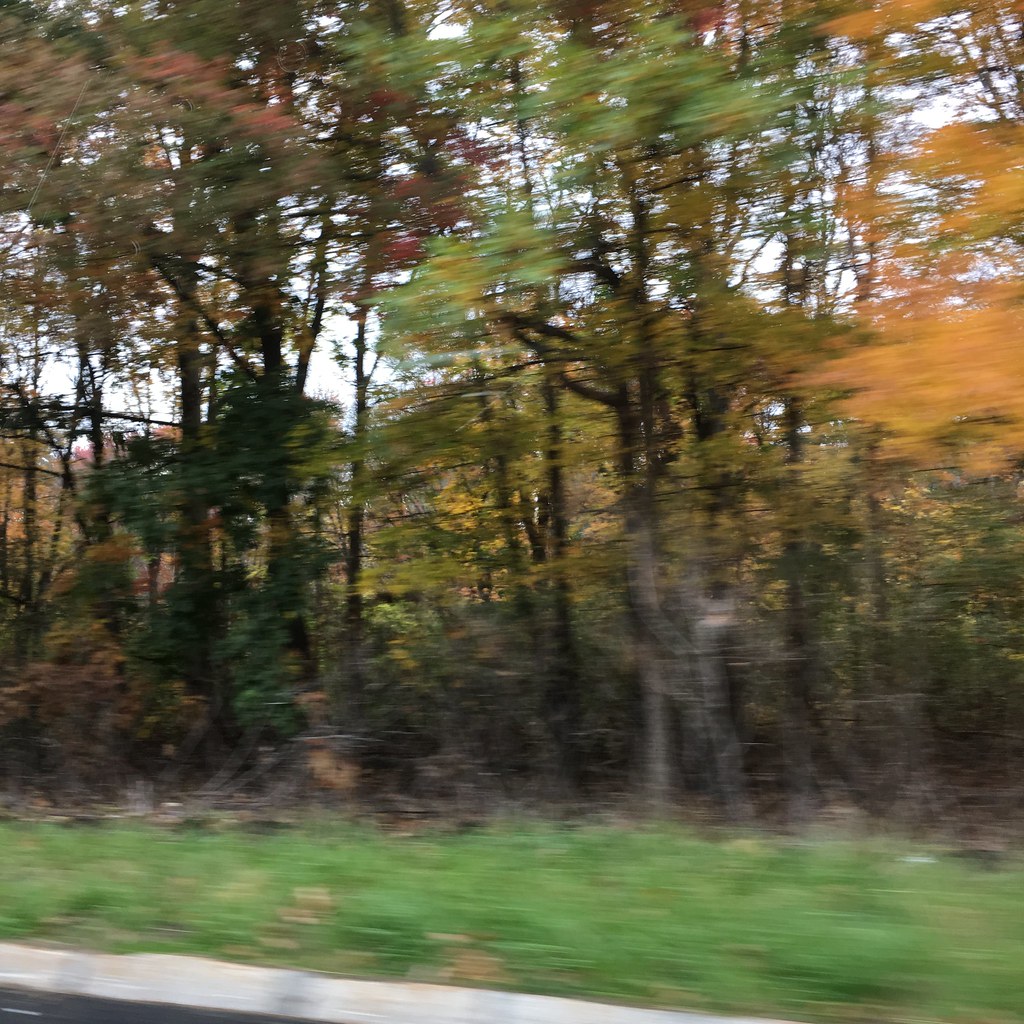Captured from the window of a moving vehicle, this slightly blurred photograph showcases a dense forest scene. In the bottom left corner, the edge of the road is visible, hinting at the motion of travel. The forest is composed of tall, slender trees adorned with a vivid spectrum of autumn foliage. The top left of the image is graced with striking red leaves, while the top right features a display of vibrant orange. Centrally, a mix of green leaves predominates, accented by hints of yellow. At the base of the photograph, tall grasses line the road, completing this picturesque view of nature's seasonal transformation.